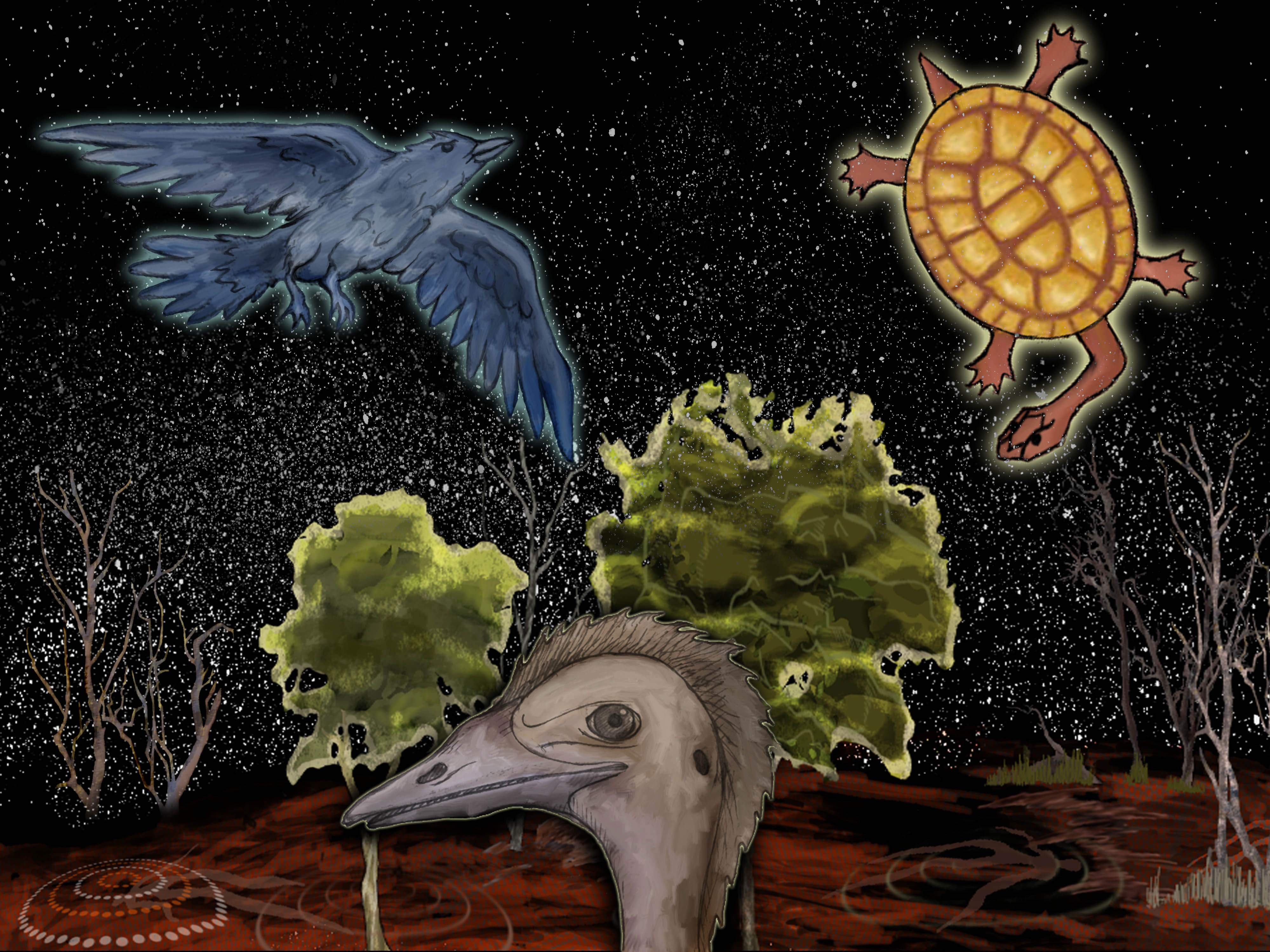The artwork, seemingly a digital rendering or stylized painting, features a dark, starlit sky filled with numerous white dots representing stars. The background consists of two leafless, weathered trees flanking the scene, their thin, bare branches reaching out as if in winter. Grounded below is a tapestry-like surface in rich red, black, and rust hues, embellished with concentric circles formed by white and orange dots, creating a geometric pattern against the earth-like tones.

Dominating the foreground is a detailed portrayal of a bird that resembles an ancient creature. This bird, possibly an ostrich or duck, has a distinctive mohawk of fuzzy feathers running from the top of its head down its neck. Its gray, elongated beak—adorned with teeth—and piercing gray eyes project an almost prehistoric visage. Framing the bird are two indistinct trees with green splotches, suggesting patches of leaves amid the barren branches.

In the top corners of the painting, two additional animals contribute to the scene's ethereal atmosphere. On the upper left, a large, blue-indigo bird, likely resembling a crow, is depicted in mid-flight with wings outspread, beak pointed upwards, and legs and tail trailing behind. On the upper right, a turtle with a gold-yellow shell segmented by orange lines captures attention. Its neck extends and bends to gaze downwards at the bird below, while its reddish-orange pointed tail complements the earthy palette.

Overall, the piece melds natural elements and abstract artistry, juxtaposing life forms and celestial bodies to create a thought-provoking, surreal landscape.